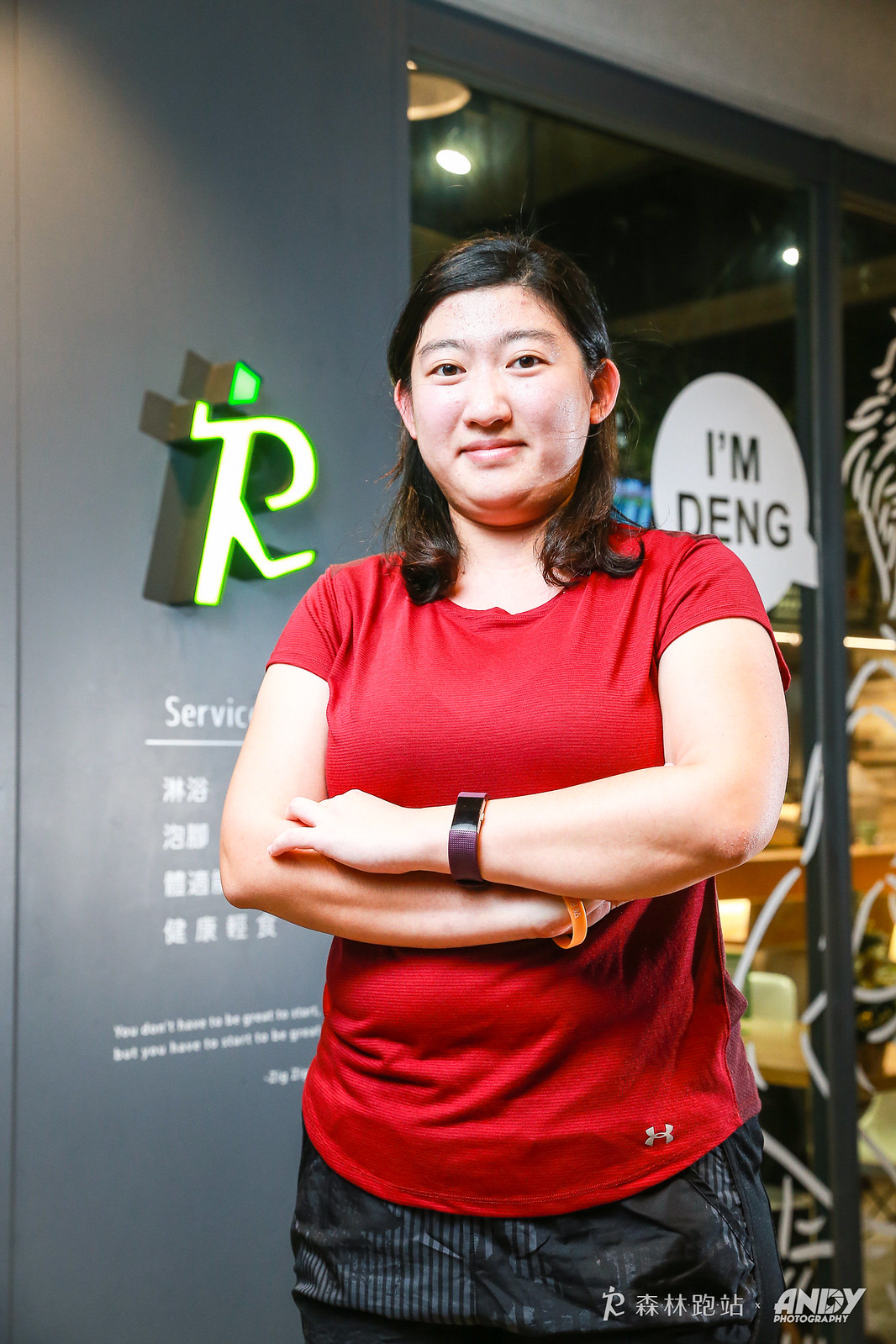The vertical rectangular photograph captures a woman standing in front of what appears to be the front of a store. She has oriental features with long, straight black hair falling to her shoulders. Dressed in a red short-sleeved t-shirt and dark-colored slacks, she exudes a sense of quiet confidence with her arms folded just below her chest. Her accessories include a black watch on one wrist and an orange bracelet on the other. The woman has a slight smile on her face as she gazes at the camera.

In the backdrop, the store's glass front is visible with various elements that add context to the image. There is a white circle with the words "I'm Deng," possibly indicating her name, as well as a fluorescent green "R" logo with Chinese writing beneath it on the wall. Indoor lighting illuminates the scene, enhancing the clarity of the photo and suggesting that it was taken inside a building. The detailed elements in the foreground and background intertwine to create a comprehensive and engaging image.